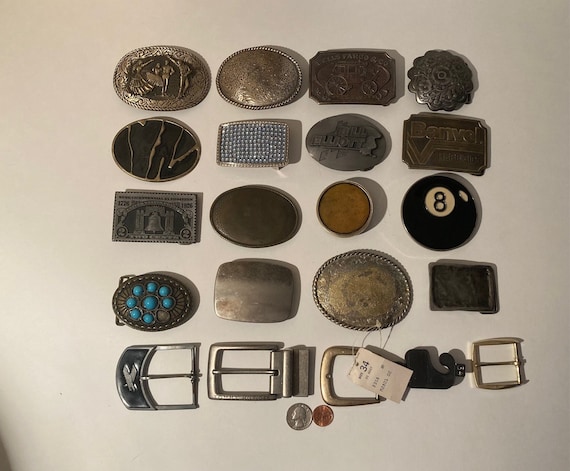The photograph captures an assortment of 20 belt buckles artistically arranged on a cream-colored background. The buckles are meticulously organized into five rows, each showcasing a variety of shapes, designs, and materials, predominantly metal with an antique finish. The top row features small metal buckles, including one shaped like a flower with embossed designs, another with a stagecoach, and an oval buckle with rust and a dancing couple framed by figures. The second row exhibits a mix of oval and rectangular buckles, some adorned with light blue to white rhinestones and intricate engravings. Especially notable is an oval buckle with a dark metal base and lighter metal designs. The third row continues with diversity, featuring an embossed rectangular buckle similar to a piece of money, an oval buckle, a fully filled round yellow buckle, and an eight-ball style black buckle. The fourth row includes a plain rectangular buckle, a metal circle with a braided edge, another large rectangular buckle, and an oval buckle adorned with turquoise pieces forming a flower pattern, with one piece missing. The bottom row displays traditional loop buckles with pins, made of different metals including simple brass, silver, goldish tones, and one with a small eagle emblem. For size context, a quarter and a penny are positioned below the buckles. Additionally, there is a price tag on a goldish buckle in the fourth row marked '34' with undecipherable text, suggesting a catalog photograph for potential purchase.